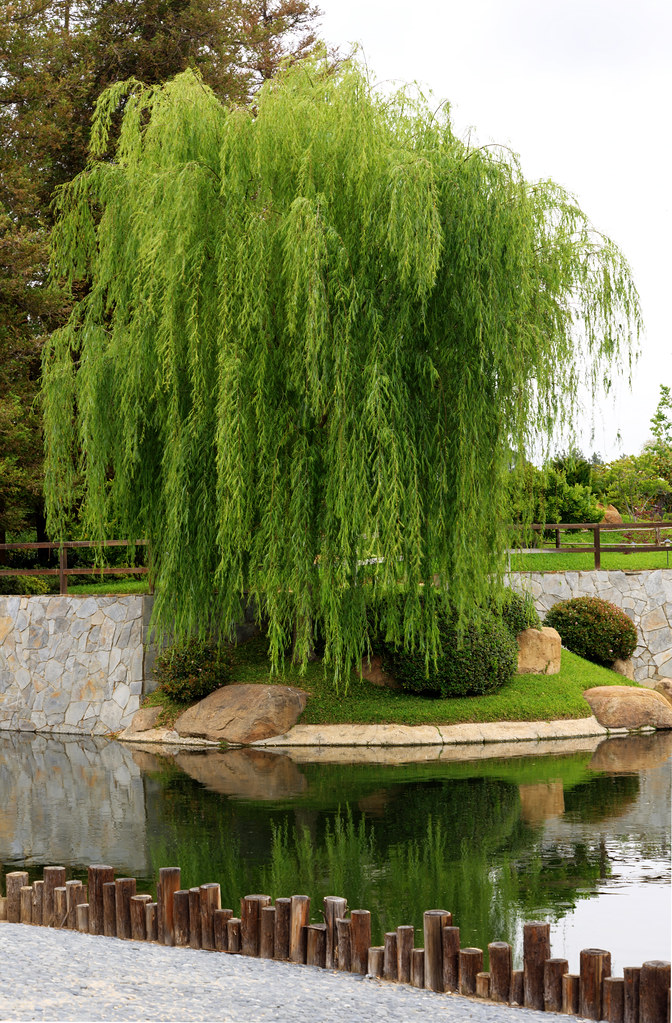The photograph captures a serene and picturesque scene in what appears to be a park or botanical garden. Dominating the composition is a brilliantly green weeping willow tree with long, mossy branches draping elegantly over a few small, round bushes. These elements are situated near a small body of water, with the tree's drooping branches partially reflected on the water's surface. In the foreground, there are numerous cream-colored rocks scattered amidst patches of grass and a short, wooden bench, providing a spot to admire the view. A cobblestone-decorated wall with a very short fence runs along the path, adding structure to the natural setting. The sky is overcast, providing a muted background that enhances the lush greenery of the scene. There are no people, animals, or visible writings in the photograph, emphasizing the tranquil and undisturbed nature of the location.